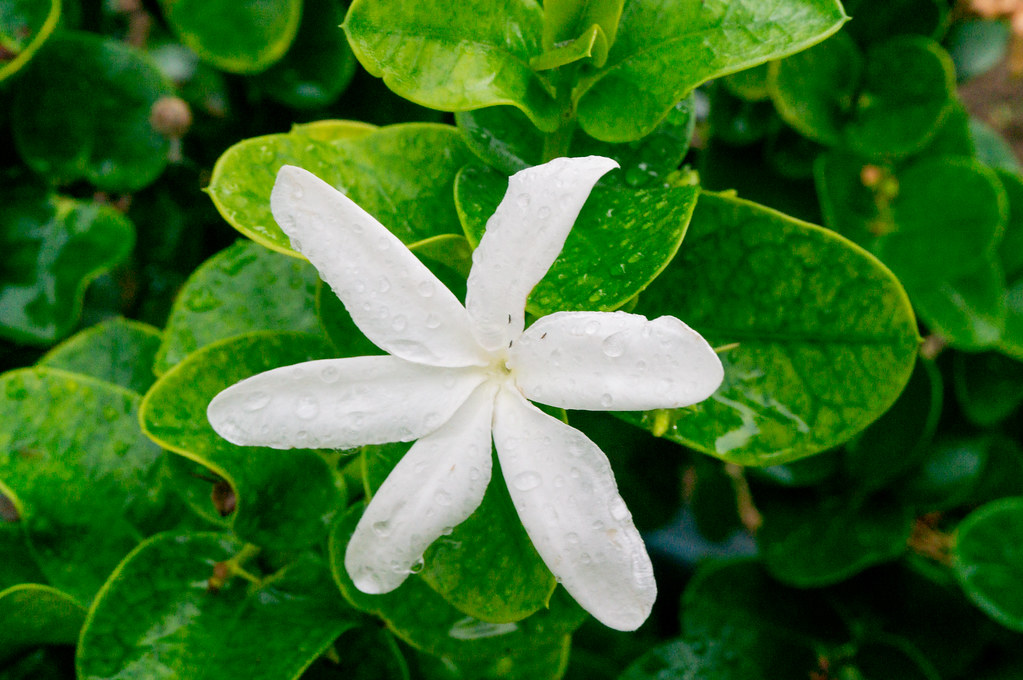This close-up photo captures a white flower with six long, thin, oval-shaped petals that taper at the center and end in gentle snub-nosed curves. The flower's core reveals intricate black stamens and pistils. Water droplets adorn the petals, adding a fresh, dewy appearance to the scene. Surrounding the flower, a cluster of rich, deep green leaves with brighter lime-green edges stretches outwards, each leaf featuring a prominent central vein and ending in a slight point. The leaves, much like the petals, are also decorated with glistening water droplets, suggesting a recent rain or watering. In the background, blurred dark green foliage provides a soft, natural backdrop. Notably, a small bud can be observed in the upper left, hinting at new growth, while a touch of brown is visible in the upper right corner. The overall composition emphasizes the delicate beauty and freshness of the flower amid lush green leaves, with a hint of nature's ongoing cycle.